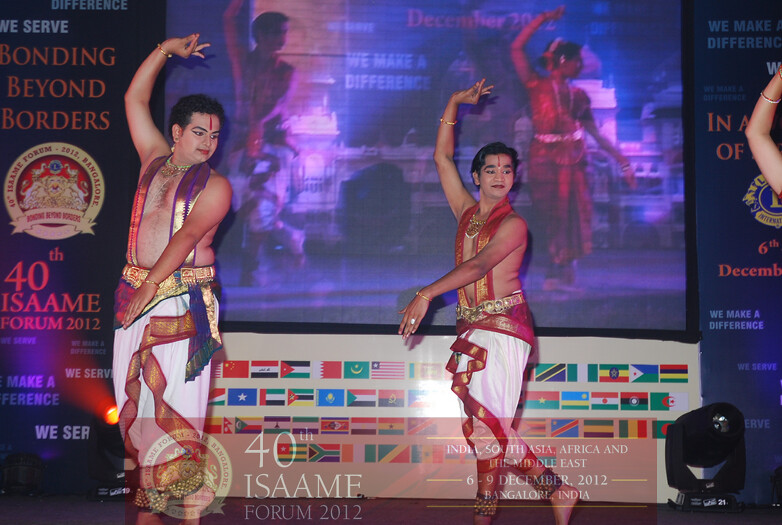Three Indian men are dancing on stage in a feminine style, characterized by fluid hand gestures and body movements. The two men at the center have gelled black hair and are seen with their right arms raised, forming a bird shape with their fingers. Their left arms hang down in front of them, and they are in a dynamic dance pose with one leg straight and the other bent at the toes. They are shirtless, adorned in gold-colored silk suspenders that connect to a gold belt, and wearing white, loose-fitting pants. Each dancer has a vertical red streak on their forehead and bracelets on both wrists. The third dancer is only partially visible, with his arm peeking in from the top right corner of the image.

The backdrop features a blue wall with incomplete text that reads "we make a difference" and dates, along with a small blue circle with a yellow ring and symbol that is too small to read. Central to the stage is a screen showing images of a man and woman in a similar dance pose, perhaps mirroring the live performers. Below the screen are flags representing around 40 countries, with the text "40th ISAAME Forum 2012" and "Bonding Beyond Borders" prominently displayed. Additional details in the background include stage lighting and rotating black spotlights, enhancing the cultural and celebratory atmosphere of the presentation.